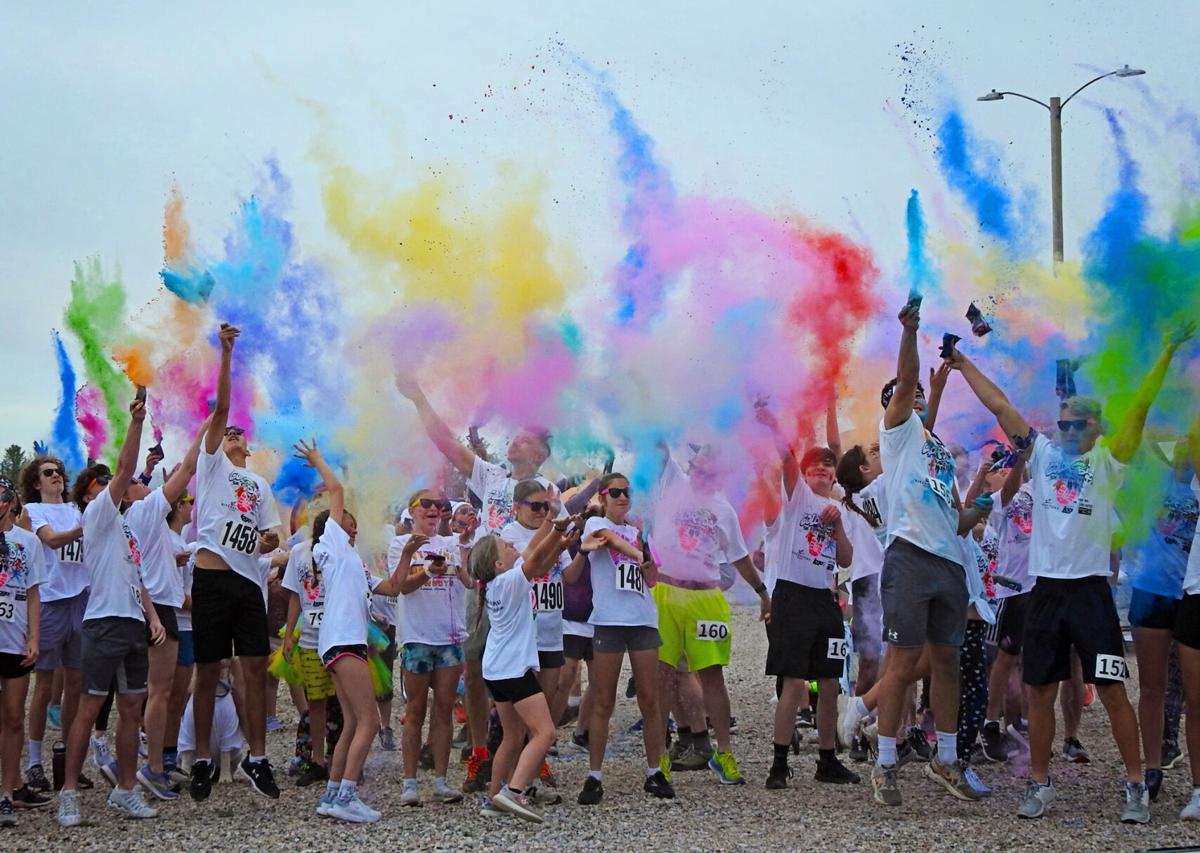The image captures a lively group of people participating in a color run, evident from their white T-shirts adorned with numbered bibs and vibrant colored powders filling the air. They stand on a gravel ground, creating a festive atmosphere with rainbow-hued plumes of powder—green, orange, blue, red, pink, yellow—shooting upwards, many released by participants' outstretched hands. The sky above is a clear blue, interrupted only by a double streetlight on the right side of the frame. A mixture of men and women, varying in age, height, and hair types—long, curly, blonde, black, brown—are depicted, many sporting sunglasses and all wearing running shoes. Notably, one individual in lime green shorts stands at the forefront, and another captures attention by jumping. The dynamic scene is further energized by numbers like 140, 148, 1458, and 160 visible on their attire, signifying their involvement in this spirited event.